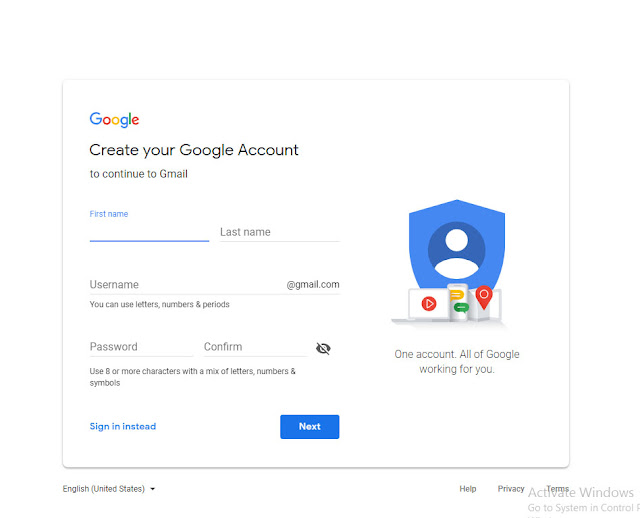The image showcases a screenshot of a Google account creation page with a white background. Prominently positioned at the top left is the iconic Google logo. Beneath it, the phrase "Create your Google Account" is presented in large, bold black letters followed by the instruction "to continue to Gmail." 

The form begins with two side-by-side input fields: "First name," which features a blue underline indicating it is in focus, and "Last name," marked by a gray underline. Below these name fields is another field designated for "Username" with "@gmail.com" appended to it, accompanied by a hint stating that you can use letters, numbers, and periods.

Next, there are two password fields placed one under the other: "Password" and "Confirm." Both fields include an "eye" icon with a strikethrough, allowing users to toggle the visibility of their typed passwords. A note beneath these fields advises using "eight or more characters with a mix of letters, numbers, and symbols."

Following this, in smaller text, there are two navigational options: a blue link labeled "Sign in instead" and a blue "Next" button for proceeding with the account creation. Adjacent to these, a distinctive blue shield icon shows a default avatar.

At the bottom of the page, a reassuring message states, "One account, all of Google working for you."